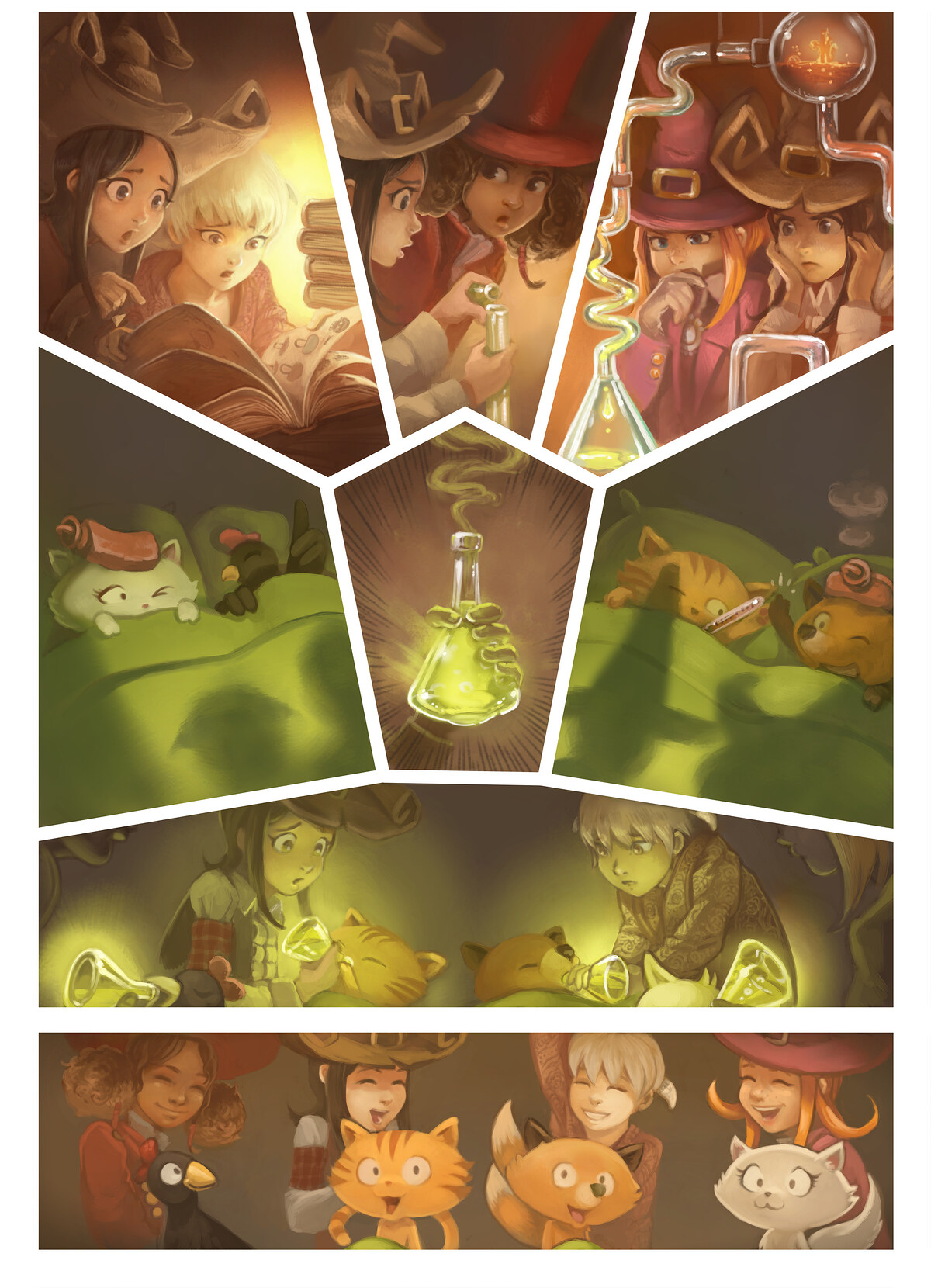The image features a series of cartoon panels depicting the adventures of two girls. Starting from the top left corner and moving clockwise, the first panel shows the two girls, one with dark brown hair and the other with blonde hair, engrossed in a book. The second panel reveals the same girls engaging in a science experiment; one wears a red top hat and the other dons a brown cowboy hat as they pour a liquid into a tube. In the third panel, the girls observe a beaker bubbling away with curiosity. The fourth panel shifts focus to two adorable animals peacefully sleeping in bed under green covers. The fifth panel depicts the girls feeding the slumbering animals with the substance from the tube. Finally, in the bottom panel, the once-sleeping animals are now awake and smiling happily, flanked by the two girls who share in their joy.